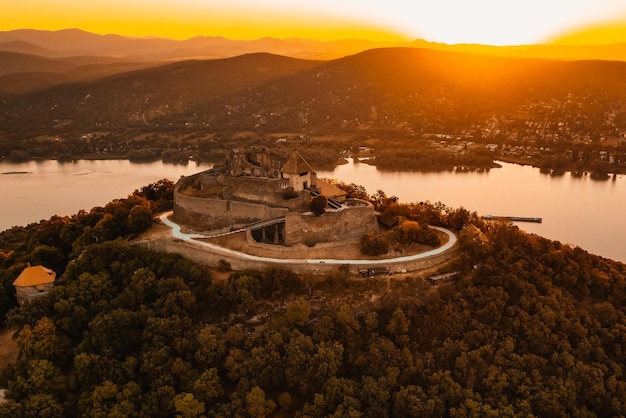An exquisite aerial photo captures the majestic Visegrad Castle, also known as the Citadel, perched atop a lush, green hill. The unique angled perspective illuminates the castle's impressive structure and reveals a serpentine pathway leading up to the fortress. The scene is framed by dense forests on the hillside and a breathtaking backdrop featuring a shimmering waterway that encircles the base of the mountain. Beyond the water, a range of mountains stretches into the distance, their dark brown hues contrasting against the bright yellow, orange, and white colors of the rising or setting sun, which casts a warm glow across the landscape. Tiny houses dot the hillsides, adding a touch of human presence to this natural and historical marvel. The entire panorama is awash in the radiant light of the sun, highlighting the intricate details of the castle and the scenic beauty of its surroundings.